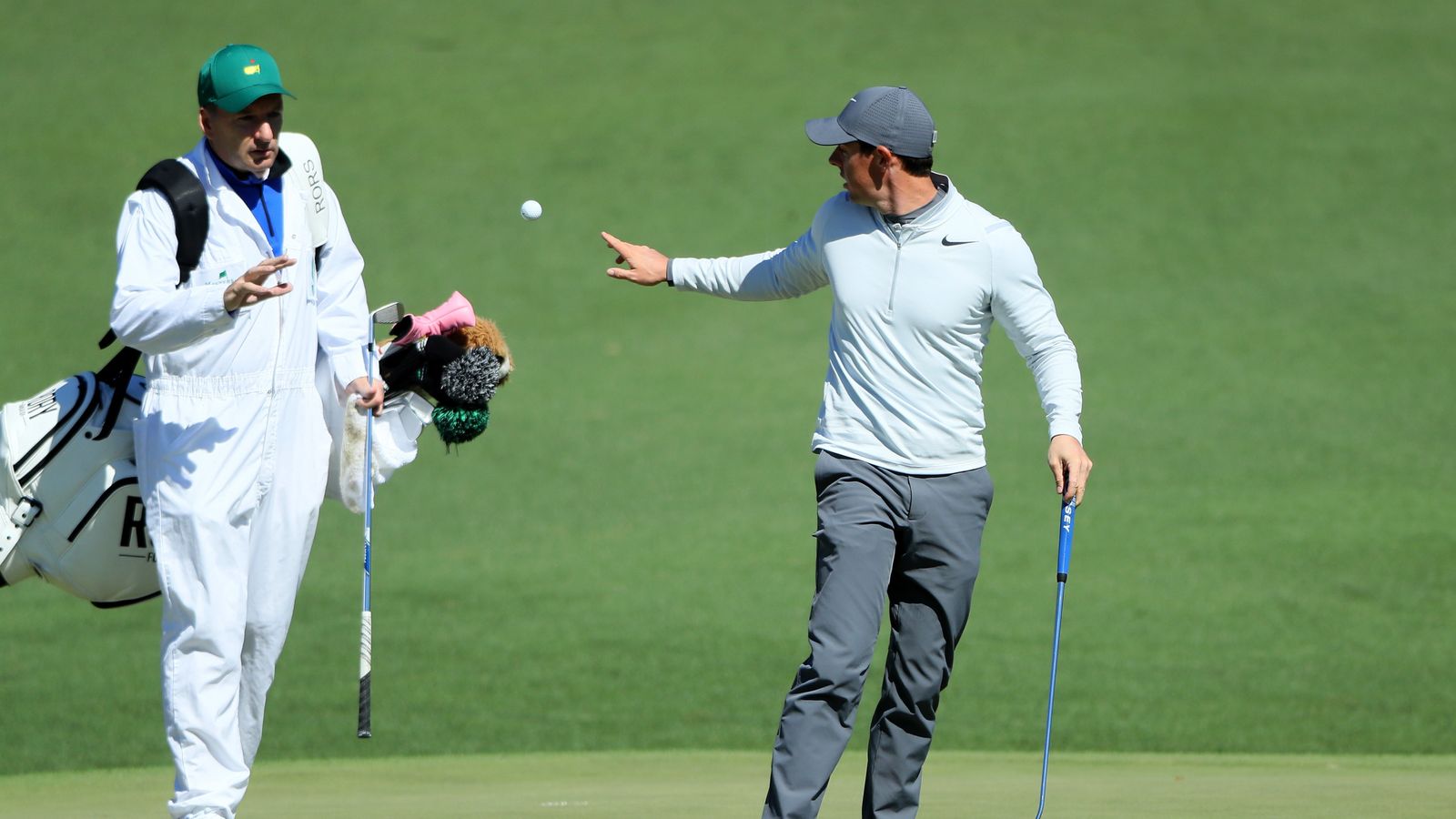In this detailed outdoor photograph taken on a golf course, two individuals are central to the scene. The first individual, resembling the professional golfer Rory McIlroy, stands prominently wearing gray pants, a white long-sleeve top with a Nike logo on the left chest, and a gray cap that slightly reveals his dark hair. He is of pale Caucasian ethnicity and is turned to the side, tossing a golf ball mid-air toward his caddy. His caddy is attired in an all-white suit with a blue shirt underneath, and a green baseball cap. He is poised to catch the ball with his right hand, while holding a golf club just below the head in his left hand. The caddy also carries a white golf bag on his shoulder, adorned with various colored socks on the clubs and an indistinct "R" marking. The vibrant green grass of the course contrasts with a patch of darker green grass in the background, capturing the essence of a bright daytime golfing scene.